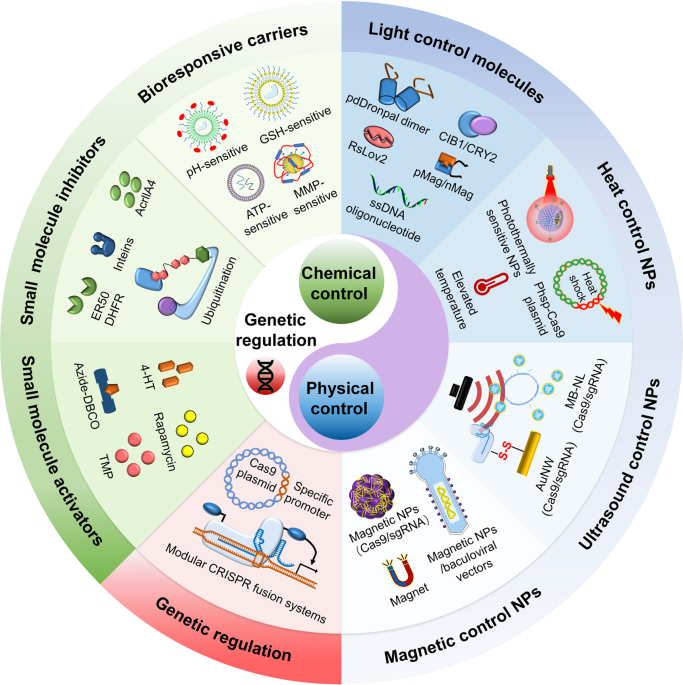This infographic embodies a vibrant, detailed circular diagram reminiscent of a pie chart, designed for professionals in the fields of biology or chemistry. At its center is a striking white and purple yin-yang symbol, representing "chemical control" and "physical control," with "genetic regulation" intricately woven within the white of the yin-yang.

The diagram is divided into eight distinct, colorful wedges, each addressing a specific area of biological control mechanisms. Starting from the top and moving clockwise, the wedges are labeled: "Bioresponsive Carriers," illustrating categories like pH sensitive, GSH sensitive, ATP sensitive, and MMP sensitive; "Light Control Molecules"; "Heat Control NPs"; "Ultrasound Control NPs"; "Magnetic Control NPs"; "Genetic Regulation"; "Small Molecular Activators"; and "Small Molecular Inhibitors." Each wedge encompasses detailed subcategories and corresponding images to encapsulate the specific types of controls and their applications.

The entire graphic is awash in vibrant hues of blue, green, red, and purple, creating an eye-catching and informative visual aid that succinctly conveys complex information about various molecular and physical control mechanisms within a single, cohesive image.